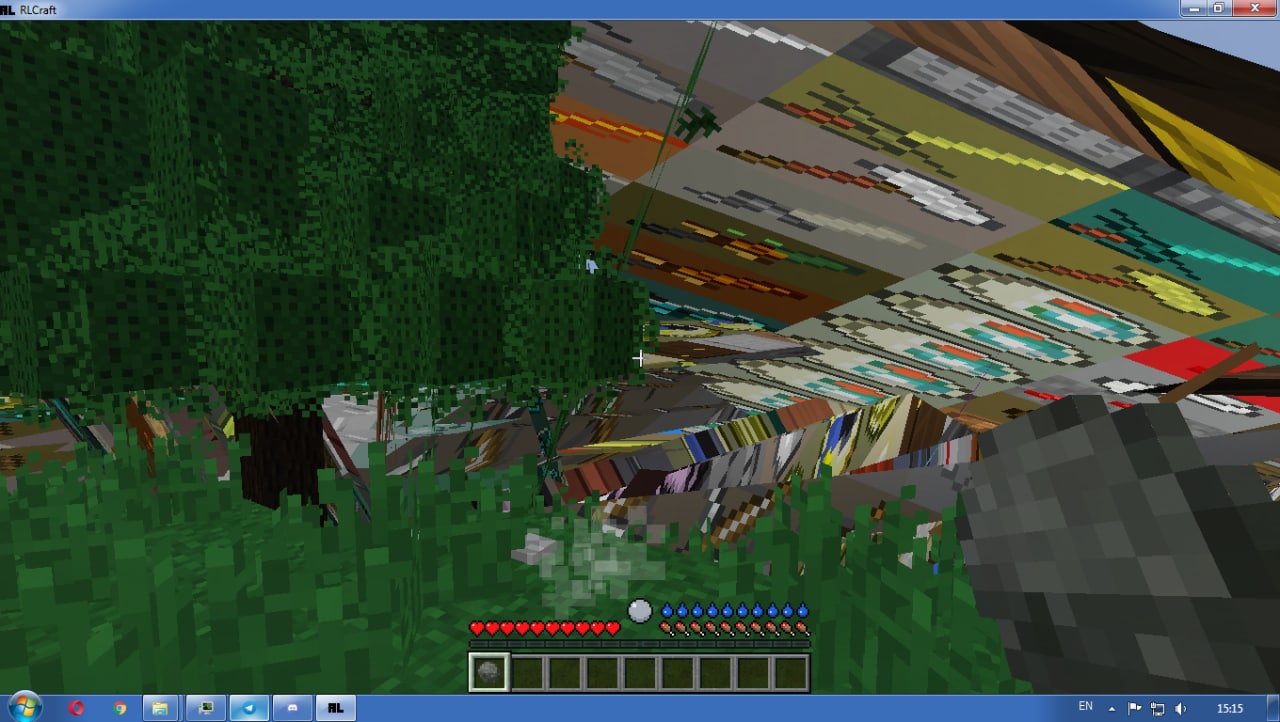This computer-generated image appears to be a frame from the video game RLCraft. Surrounding the game window are the blue navigation bars of the computer interface. The top bar features the game title "RLCraft" on the left-hand side and standard window controls (minimize, maximize, and close) on the right-hand side. The lower bar includes the iconic Microsoft logo in red, green, blue, and yellow, along with various navigational icons for open tabs such as files and other applications. The time is displayed as 15:15 on the lower right corner, accompanied by several other system icons.

The game view is distorted and captures an overhead perspective of a green field next to a castle-like wall or fence adorned with intricately designed, colorful panels in greens, yellows, whites, and oranges, some resembling Indian-style shields. At the base of this wall, there are small character figures visible. The player’s score is indicated by red hearts on the left and blue teardrops on the right, suggesting health and possibly a secondary metric within the game.